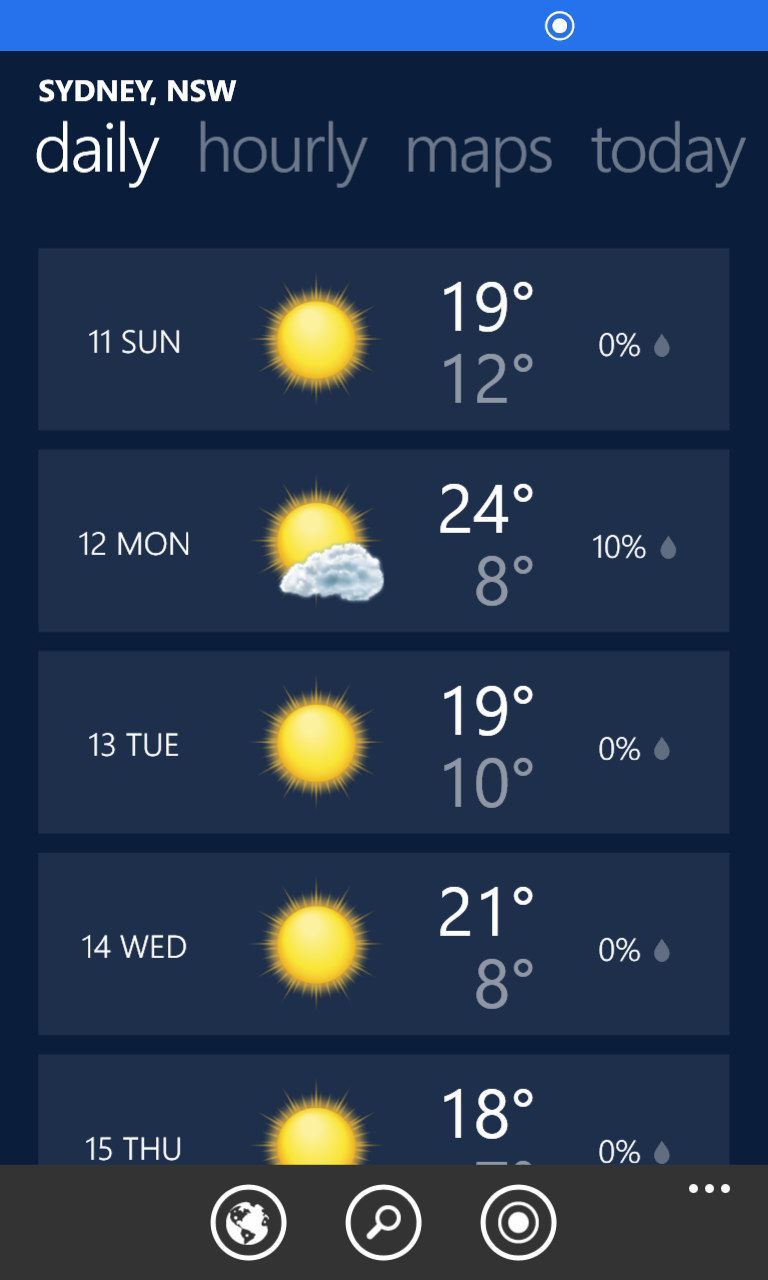The image is centered around weather information for Sydney, NSW. At the top, "SYDNEY" is prominently displayed in uppercase letters, followed by "NSW." Beneath this, the word "DAILY" is highlighted in bold white print. Below, "Hourly Maps" and "Today" are also displayed. 

The weather forecast spans from the 11th to the 15th, presented as follows:

- **11th (SUN, Sunday):** Full sun with a high of 19°C and a low of 12°C.
- **12th (Monday):** Full sun with a cloud icon, high of 24°C, low of 8°C, and 10% precipitation.
- **13th (Tuesday):** Full sun with a high of 19°C and a low of 10°C.
- **14th (Wednesday):** Full sun with a high of 21°C and a low of 8°C.
- **15th (Thursday):** Full sun with a high of 18°C and 0% precipitation, visually represented by a raindrop icon.

The image effectively showcases a weeklong weather forecast for Sydney with clear and precise details, including temperature highs and lows, sun/cloud symbols, and precipitation percentages.